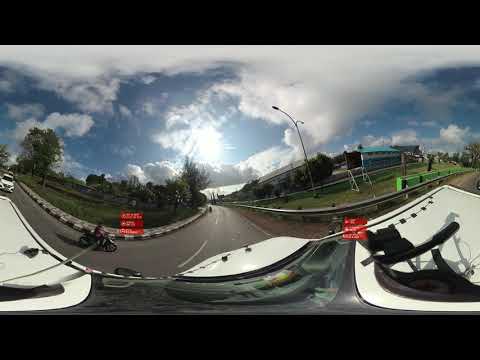This image, captured with a fisheye lens, presents a slightly distorted panoramic view of a daytime outdoor scene. The sky, occupying the top half of the image, is vivid blue, adorned with large, puffy white clouds and a bright sun at the center. 

The scene below features a long, winding road that meanders through the frame, intersecting at multiple points. This road has metal railings on one side and a wooden fence on the other, each lined with lush green trees. On the left side of the road, there's a person riding a motorcycle and an oncoming white vehicle. A teal-colored building and a streetlight are visible further along this side. A soccer net is set up near the road, nestled among the trees.

On the right, there is another segment of the road that curves upwards and towards the right, leading into a hilltop. A large building can be seen perched on this hill. The fisheye lens gives the image a unique distorted effect, adding to the intrigue of the scene.